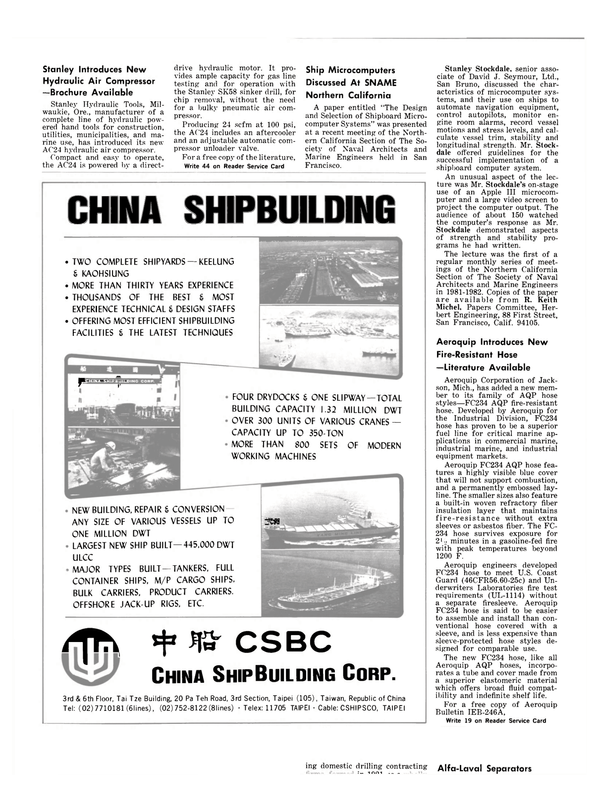The image is a vertical, black-and-white newspaper page, dense with black type on a white background, divided into distinct columns and sections. Prominent headlines include: "Stanley Introduces New Hydraulic Air Compressor, Brochure Available," "Ship Microcomputers Discussed at SNAME, Northern California," and "Aeroquip Introduces New Fire-Resistant Hose, Literature Available." These articles discuss innovations in shipbuilding technology and related equipment.

The most substantial section is an advertisement for China Shipbuilding, occupying much of the left side of the page. This ad highlights two complete shipyards with over 30 years of experience in the industry, showcasing their capabilities in constructing, repairing, and converting various vessels. It details the facilities available, including dry docks and crane capacities, and features photographs of completed ships, the shipyards, and workers actively building ships. Contact information for China Shipbuilding Corporation, including address, telephone, and TELEX number, is provided at the bottom of the advertisement.